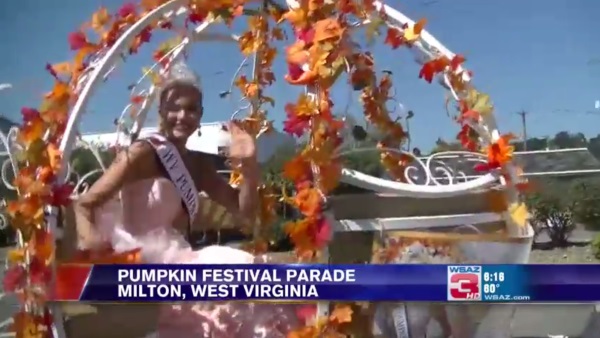The image is a detailed screenshot from a newscast featuring a Pumpkin Festival Parade in Milton, West Virginia, as indicated by the bottom banner. The news channel's logo reads either WBAZ or WSAC Channel 3, depending on different interpretations, and includes the time and temperature, which are either 818 o'clock, 80 degrees, or slightly different temperatures provided by other sources. 

Central to the image is a young, thin blonde woman wearing a crown and a pink, ruffled dress with a sash that likely says "Miss Pumpkin" or similar, suggesting she is a festival queen or prominent figure in the parade. She is riding a ornate float designed to resemble a pumpkin carriage with exposed ribs, decorated with orange and red fall foliage, creating a very autumnal scene. The float is constructed with a white trellis-like structure covered in autumn leaves. She is smiling and waving toward the camera, conveying a sense of joy and festivity. The background is blurred, adding a sense of motion to the parade scene, and the sky is vividly blue, enhancing the vibrant, celebratory atmosphere. No other people are visible in the image.